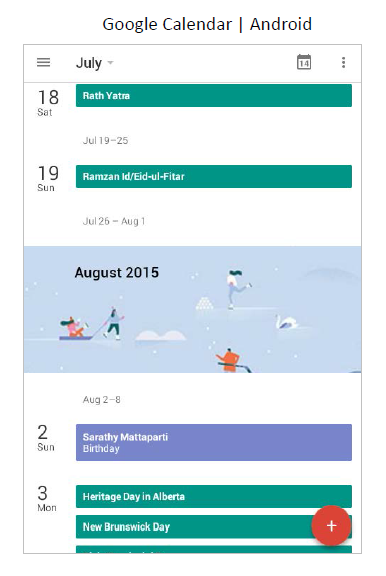A screenshot of the Google Calendar app on an Android device displays a detailed view of various dates and events. At the top, the header reads "Google Calendar Android." Below the header is a white box outlined with a gray border. In the upper left corner of the box, there is a hamburger menu icon. Next to it, the current month "July" is displayed, accompanied by a calendar icon and the date "14". In the upper right corner, a vertical ellipsis (three dots) icon is visible.

The main content of the calendar begins with "July 18, Saturday" followed by an event highlighted in a turquoise box labeled "Rathvate" (the text is slightly blurry and hard to read). Below this, the calendar continues with "July 19-25," featuring "July 19, Sunday" and another turquoise box for the event "Ramzan, I-D-O-V-T-A-R."

The calendar then spans "July 26 - August 1," transitioning to show an image of people ice skating and pulling a sled beneath this section. Underneath the picture, the calendar displays "August 2015," followed by "August 2-8" with a note for "August 2, Sunday," indicating it is "somebody's birthday."